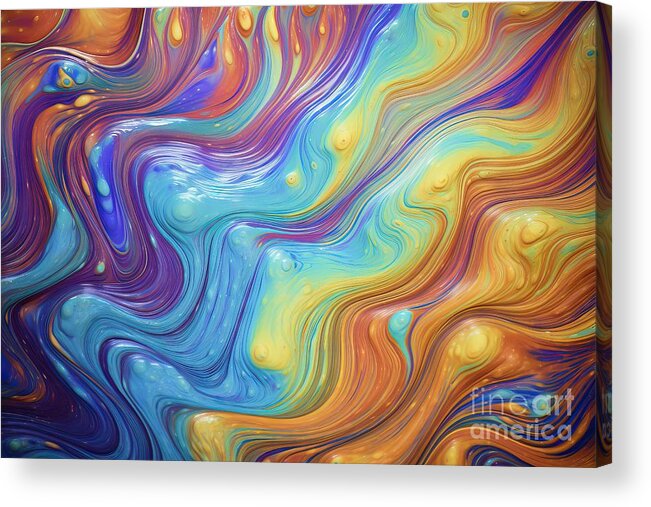This modern art piece, referencing Fine Art America in the lower right corner, is a vibrant abstract painting characterized by its squiggly, uniform lines that generally flow diagonally from the upper right to the lower left. The color palette is rich and diverse, featuring shades of light blue, yellow, orange, red, and purple, which bleed together seamlessly. The painting evokes a sense of motion, reminiscent of oil swirling in water, and includes small, bubble-like elements dispersed throughout the canvas. The center prominently features a vibrant blue that transitions into purples, yellows, and oranges as it moves towards the bottom right. The canvas edges are visible, suggesting it is a canvas piece that slightly protrudes from the wall. The artwork is set against a white background, offering no additional contextual environment, and no artist's inscription is present.